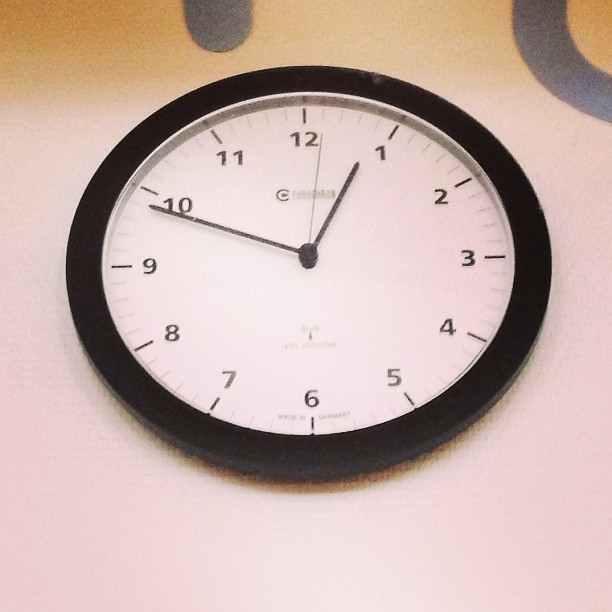This photograph showcases a circular wall clock mounted against a background that appears to be an off-white wall or possibly a tarp. The clock features a white face encircled by a black border approximately one inch thick. The numerals and hands, including the second hand, are all black, providing a stark contrast against the white background. The time displayed on the clock is 12:51 and one second, with the second hand positioned just past the 12 o'clock mark.